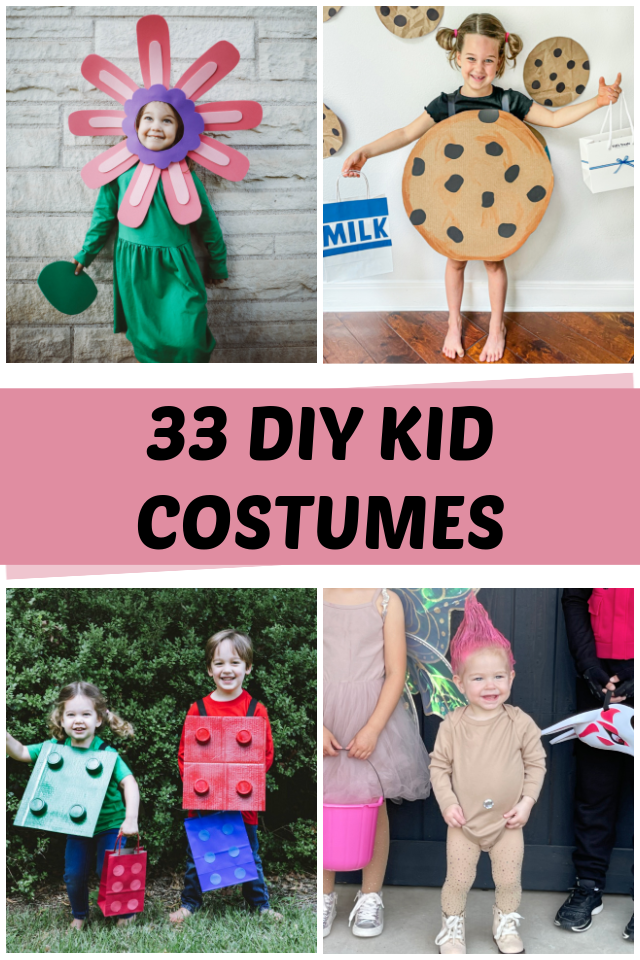This image consists of a collage of four photos, organized in a two-by-two grid, featuring children in various DIY costumes. At the center of the collage, a pink rectangle with black bubbly capital letters reads "33 DIY Kid Costumes." 

In the top left photo, a small child is dressed as a flower, adorned with pink paper petals around their head and a purple center. The child wears a green dress and is positioned against a gray wall. 

The top right photo showcases a young girl dressed as a chocolate chip cookie. She wears a cookie-shaped overall dress over a black shirt and t-shirt, and holds a paper bag labeled "milk." She stands barefoot against a gray backdrop decorated with cookie drawings.

The bottom left image features two children dressed as Legos. The girl wears a green shirt and blue pants with a blue Lego piece hanging around her neck and carries a matching bag. Beside her is a boy in a red shirt and jeans, with a red Lego piece and a blue bag. They are positioned outdoors with plants in the background.

The bottom right photo depicts a toddler in a beige long-sleeve onesie with spiked pink hair, resembling a troll doll. The scene includes another girl in a brown dress holding a purple bucket, and part of a person in a red shirt and black pants holding a red and white mask.

This diverse array of costumes showcases creative, homemade ideas suitable for kids, embodying fun and imagination.